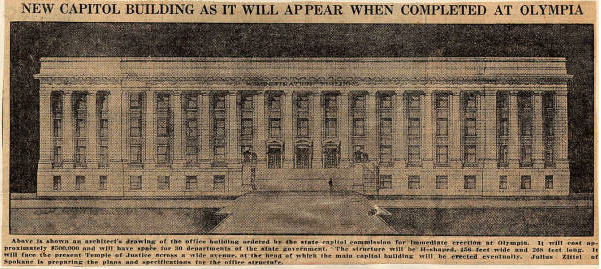This is an image of an old newspaper article featuring an artist's rendering of the future Capitol building in Olympia. The headline reads, "New Capitol Building as it will appear when completed at Olympia." The article is printed on a yellowed, tan background with black text. The central artwork showcases a long, rectangular building with a flat roof, resembling the structure seen on the back of a dollar bill. 

The building is characterized by its numerous pillars spanning from the ground to the roof, giving it a grandiose appearance. Large steps lead up to three prominent, arched doorways at the center. In front of one of these doors is a small, illustrated figure of a person, adding a sense of scale. The façade features an abundance of windows, too many to count, enhancing the building's formal and authoritative look. At the bottom of the article, a caption notes that the illustration is an architect's drawing commissioned by the state capital commissions, estimating the building's cost at approximately $500 and detailing that it will house 30 state government departments. The background of the image is very dark, making the building structure stand out prominently.